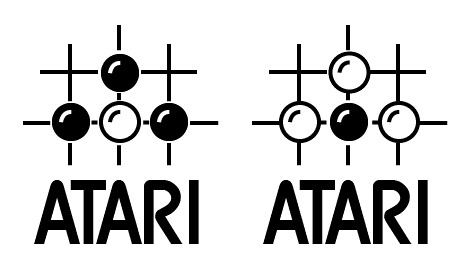In the image, the left half mirrors the right half but features different colors. The right half is in black and white, displaying the Atari logo with intersecting lines forming a grid of three vertical and two horizontal segments. At the intersections, three white circles with black lines inside sit at the top, right, and left positions, while the center circle is black with a white line inside. Below this arrangement, the word "Atari" is written in black.

The left half of the image features the same design but with inverted colors. Here, the center circle is white with a black line, while the top, right, and left circles are black with white lines. The background of the left half is white, providing a stark contrast. The same "Atari" text appears in black at the bottom of this side. The entire composition showcases these two variations of the Atari logo side by side.